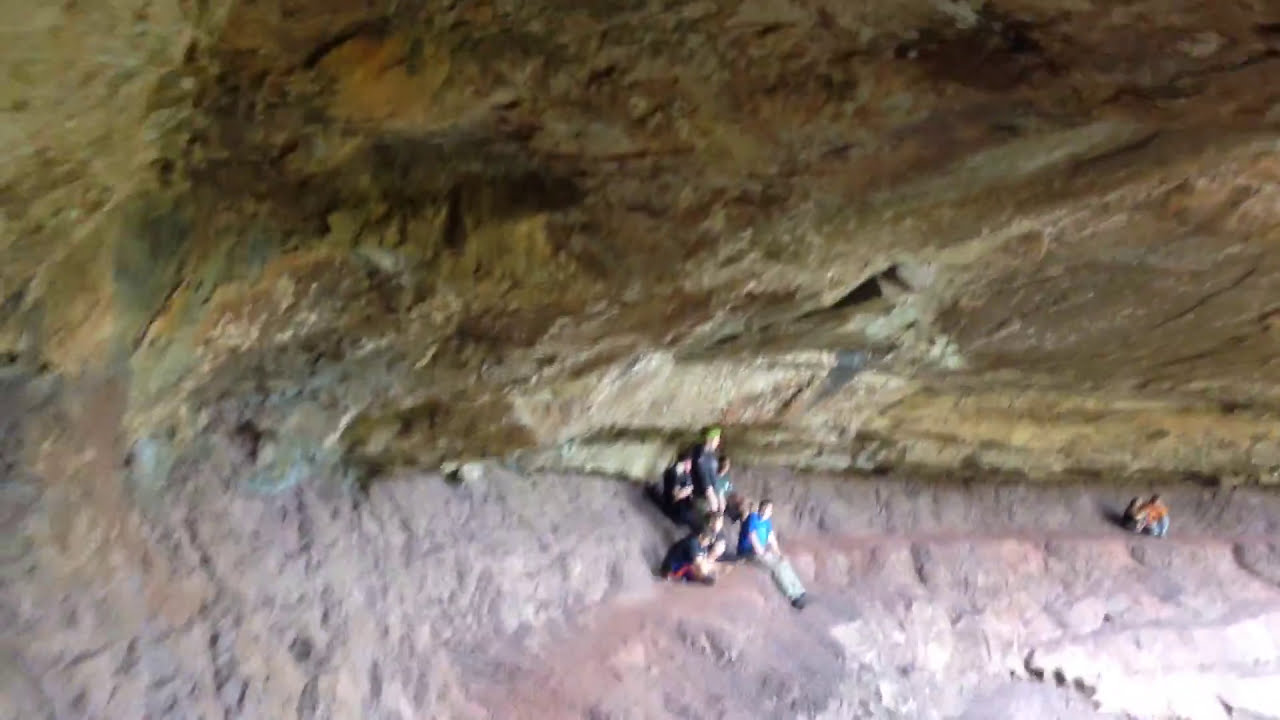This aerial photograph captures a rugged, rocky terrain, dominated by a steep cliff edge that extends down to a rocky floor below. The scene below features a small human presence, providing scale to the vastness of the rock formation. A lone individual in an orange shirt and blue pants sits on the right, seeming to enjoy the serene environment. To the left and slightly nearer, a small group of people, possibly an adult and two children, sit together in casual attire, including pants and t-shirts, appearing relaxed. The rock below them is predominantly gray with a pinkish hue, while the overhanging ledge above displays richer tones of red, brown, and orange. The rocky area appears to be solid and stable, with a notable absence of loose gravel, suggesting it could be part of a tourist-friendly cave or an outdoor natural formation. The overall composition highlights the earthy tones of the rocks and the small yet significant human elements that add context and scale to the grandeur of the scene.